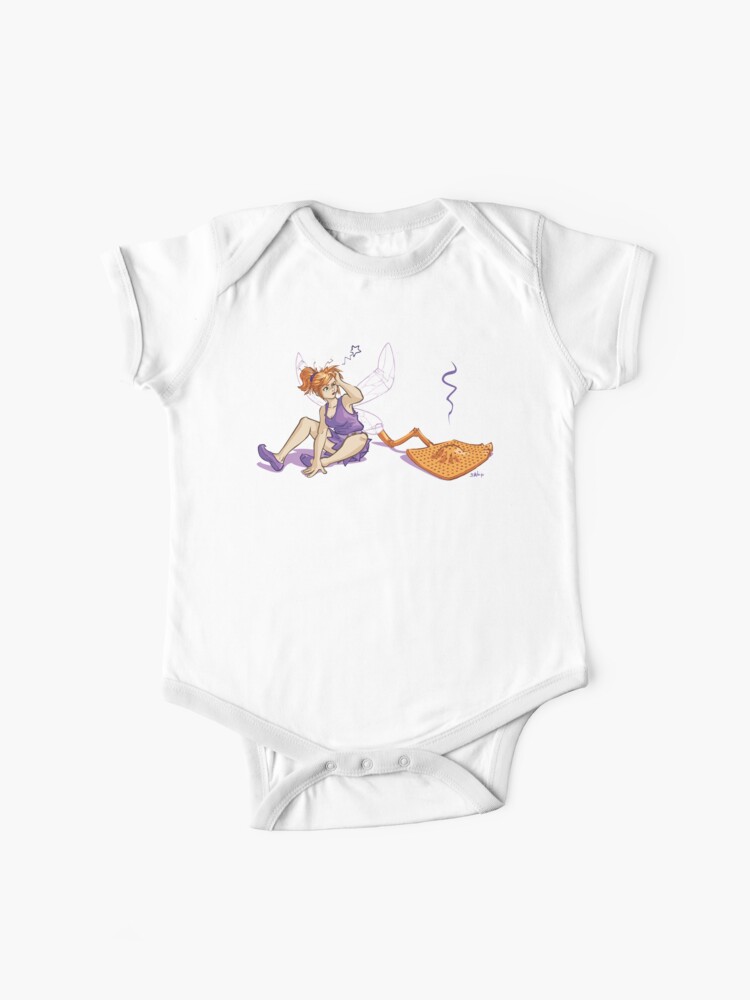The image showcases a white baby's onesie set against an entirely white background. Adorning the front of the onesie is an illustration of a fairy with pale wings and red ginger hair. The fairy, dressed in a purple outfit with matching shoes, appears slightly annoyed as she sits on the floor. Her hat, which matches the color of her hair, has fallen off. Adding to the scene, a small star emanates to depict a dazed expression. Next to her lies a broken fly swatter, suggesting an accident or mishap. The fairy's wings are bent, hinting at possible damage from the fly swatter, which may have struck her or another object.